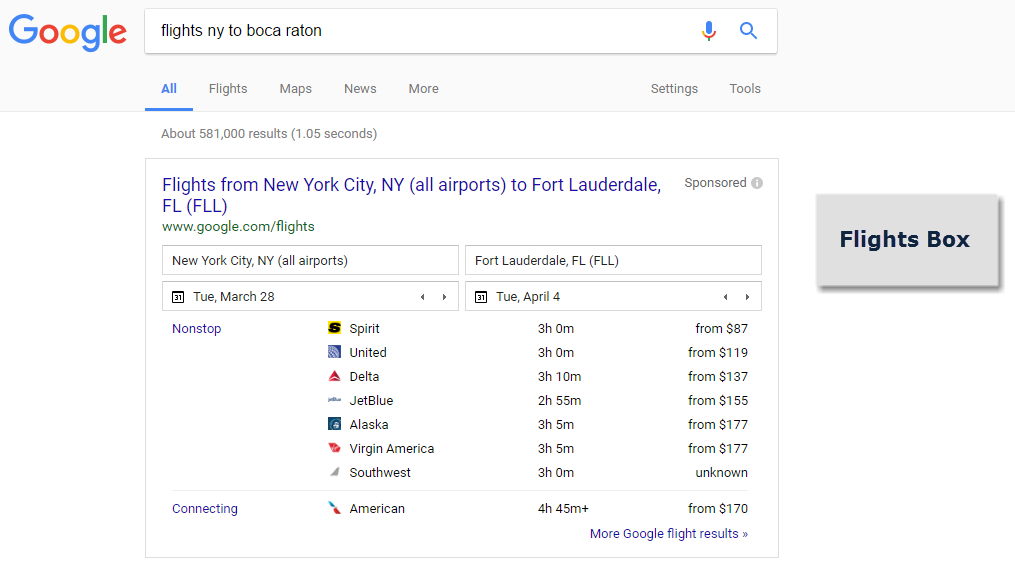The image displays a screenshot of a Google Flights search results page. At the top, there is a very light gray rectangle containing the Google logo, which is composed of letters in various colors, positioned on the left-hand side. Adjacent to the logo is a search bar with a white background, showing the query "Flights NY2 Boca Raton." To the right of the search bar, there are two icons: a microphone and a magnifying glass.

Below this strip, the interface shows navigation tabs with "All" in blue and underlined, followed by "Flights," "Maps," "News," and "More." On the far-right side are options labeled "Settings" and "Tools." Directly beneath this navigation bar is a white section that mentions the number of search results, although the exact figure is unclear, and includes some text in parentheses.

The primary content area features a white box with a gray outline. Inside, bold blue text reads "Flights from New York City, NY (all airports) to Fort Lauderdale, FL (FLL)," with a URL displayed in green underneath it, and the word "Sponsored" located at the upper right-hand corner of the box. There is a small circle icon and text indicating the origin and destination: "New York City, NY (all airports)" and "Fort Lauderdale, FL (FLL)."

Following this, the interface includes two additional white boxes, each showcasing a calendar icon. The first displays "TUE, March 28" with left and right arrows for navigation. The second similarly includes "TUE, April 4" with corresponding navigation arrows.

On the left side, the text "Non-Stop" appears in purple, and further down, also in purple, it says "Connecting." The main body lists various airlines along with flight times and prices. At the bottom, the text "More Google Flights Results" in blue is accompanied by a right-pointing arrow.

The page also contains a gray box with a darker gray shadow effect, labeled "Flights Box," completing the interface description.